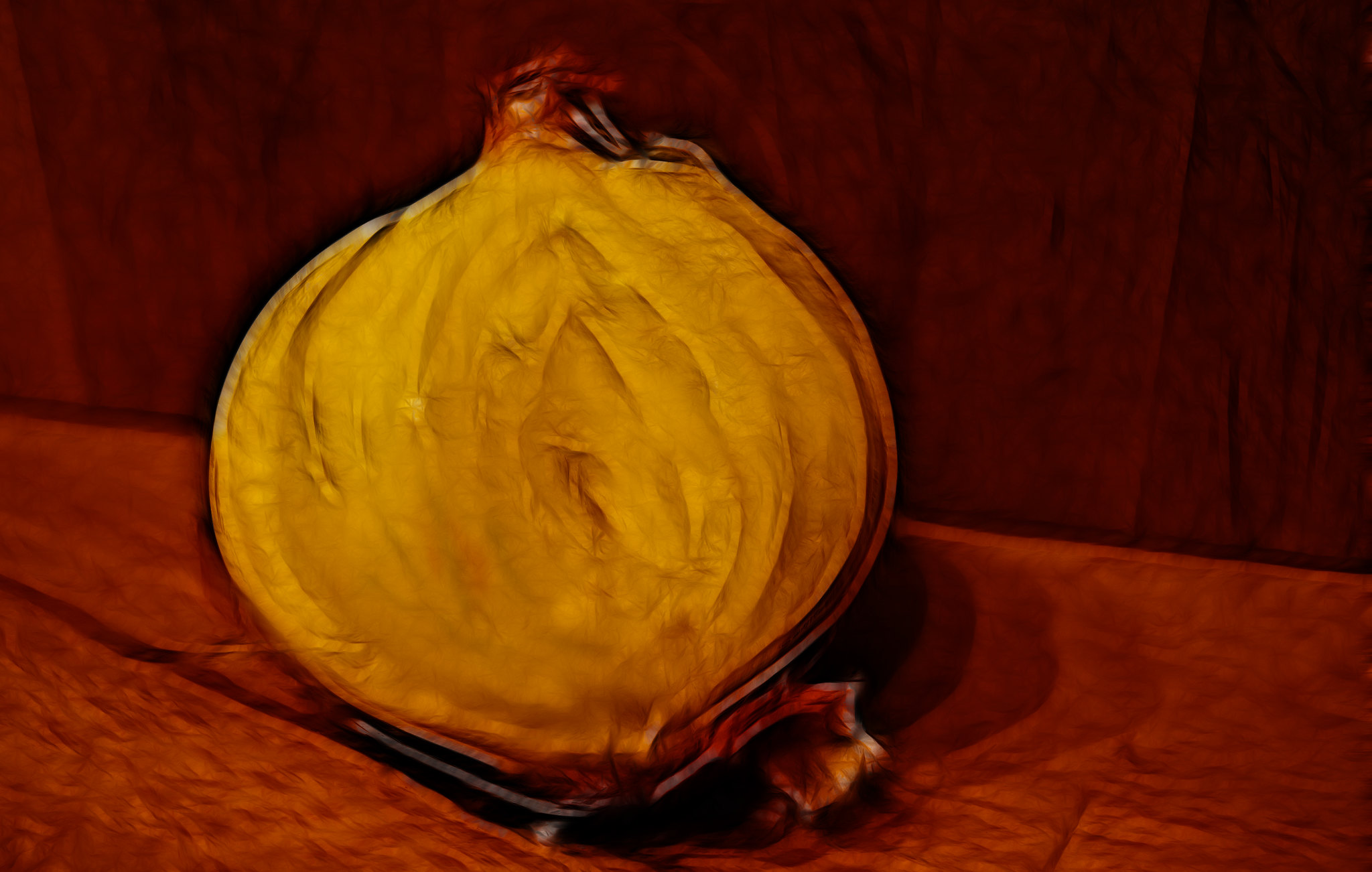The image depicts a yellow and red onion, peeled and resting on a wooden surface. The scene appears to be either an artistic painting or a photograph with a filter, giving it a slightly distorted and surreal appearance. The setting features a dark brown wooden wall and a reddish-brown floor, all rendered in a cohesive brown hue. The onion is centrally placed, showcasing its round shape with a pointed bottom and a small stem-like top. You can observe the layers within the onion starting from the center and curving outwards. The entire composition emphasizes the onion, with its peeling skin adding texture and detail, against the simplistic background, enhancing the impression of an isolated still life study.